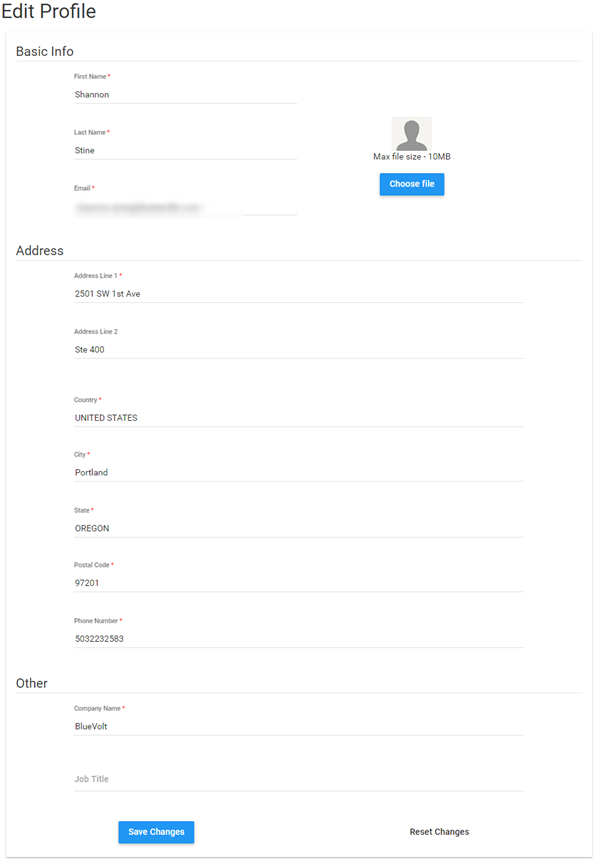The screenshot appears to be from a tablet showing a "Edit Profile" page. At the top left corner, the largest font clearly reads "Edit Profile". The page is divided into three editable sections. The first section, labeled "Basic Info," includes fields for first name, last name, and email address. The second section, titled "Physical Address," comprises Address Line 1, Address Line 2, country, city, state, zip code, and phone number. The third section, named "Other," asks for the company name and job title. At the top right, next to the Basic Info section, there is a "Choose File" button for uploading a profile photo. At the bottom of the page, there are two buttons: a blue "Save Changes" button on the left and a "Reset Changes" button on the right.